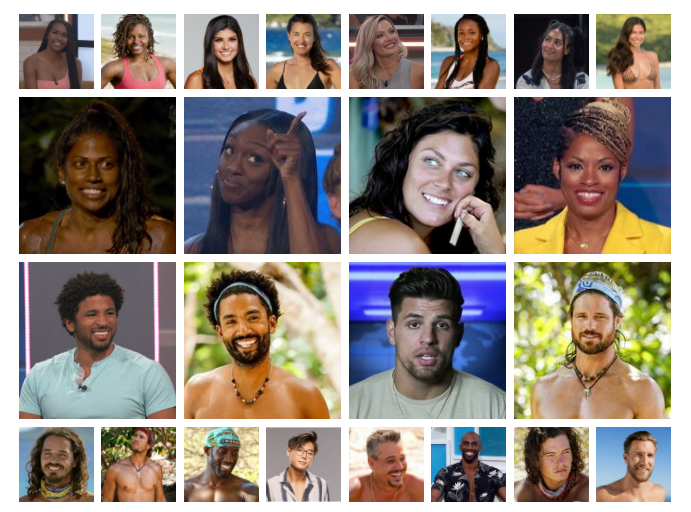The image is a detailed mosaic comprising 24 individual headshots featuring a diverse group of young, attractive contestants, likely from a reality TV show. The layout is structured with eight smaller photos in the top row, eight smaller photos in the bottom row, and two middle rows containing four larger photos each. The upper half exclusively displays females, while the lower half shows only males. Among the women, there are both Caucasian and African-American individuals, with attire varying from swimsuits to sporty clothes. One notable female is wearing a yellow jacket. Similarly, the men, many of whom are shirtless, are captured from the chest up, appearing youthful and well-built. The contestants represent various races, predominantly white, Hispanic, and African-American, suggesting a diverse cast possibly from an American show like "Survivor" or "Big Brother." The backgrounds hint that many photos were taken outdoors.